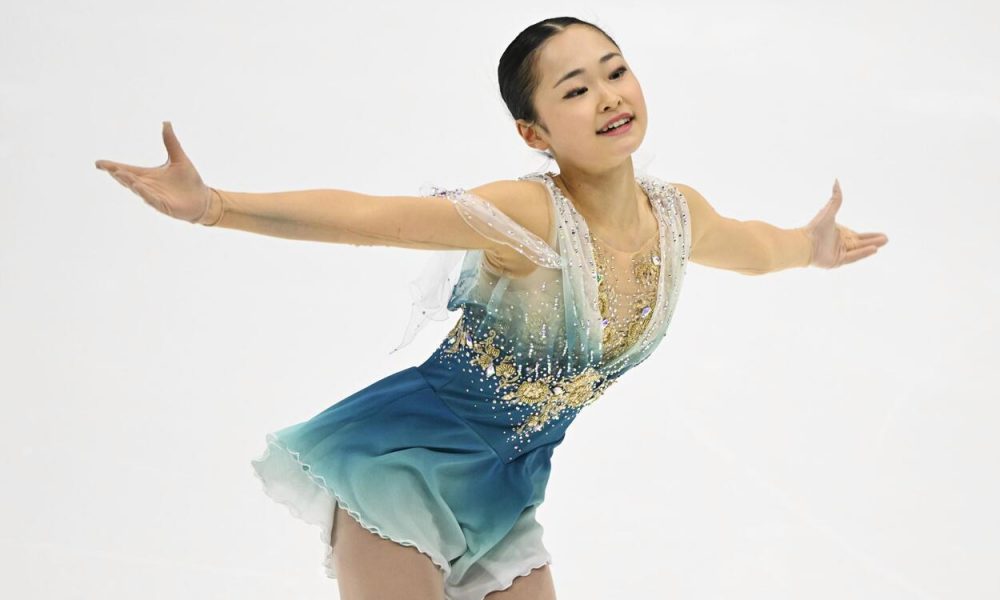This image features Michelle Kwan, the renowned figure skater, depicted from the top of her head to the middle of her thighs, with her feet and legs not visible. She is wearing a stunning blue figure skating costume, heavily adorned with intricate gold ornamentation and designed to appear as a halter top with a flowing skirt that fades to white at the hem. The costume's long sleeves match her fair skin tone, creating an illusion of bare arms, complemented by a delicate mesh inlay over her chest. Michelle's dark, glossy hair is parted in the middle and pulled back smoothly into a sleek bun. She showcases a gentle smile, revealing her upper teeth, while her dark eyes reflect her focused demeanor. With her slender arms outstretched on either side, she appears to be gliding gracefully on the ice, embodying elegance and poise.